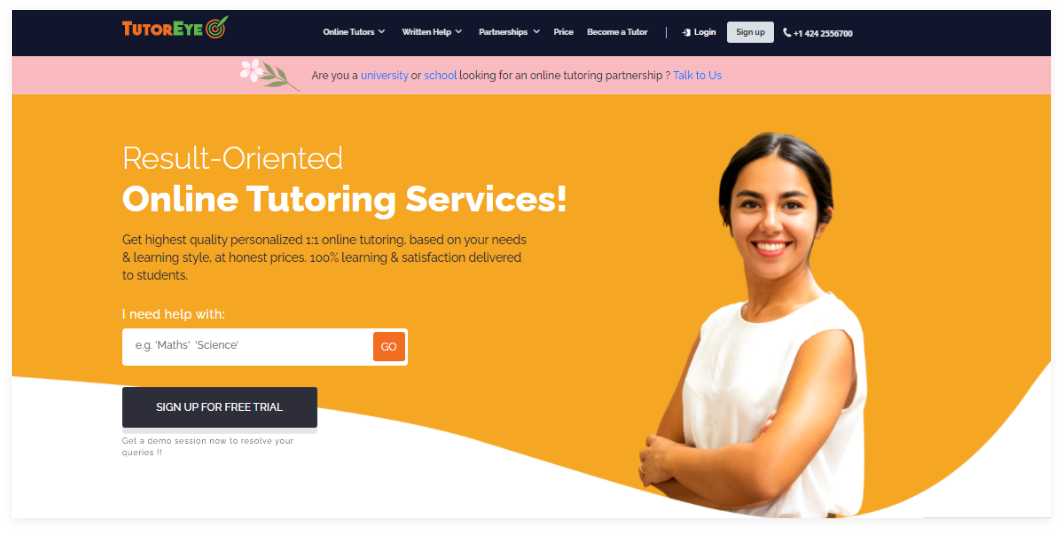The webpage presents an educational platform with a sleek design. Encased within a solid black top navigation bar, the site's branding features the word “Tutor” rendered in an orange font, seamlessly merging into “EYE” in green, accompanied by a logo—a target with intersecting orange and green elements and a green dart at its center.

Spanning rightward across the navigation bar, the following menu options, each accompanied by a drop-down arrow, are listed in white font: “Online Tutors,” “Written Help,” and “Partnerships.” Additional options include “Price,” “Become a Tutor,” “Login,” and a prominently displayed “Sign Up” button, the latter distinguished by a white-background button. Further to the right, a telephone icon is paired with the contact number “1-424-255-6700.”

The subsequent banner section is accentuated with a thin pink underline. Adjacent to a small flower graphic, the banner reads, “Are you a university or school looking for an online tutoring partnership? Talk to us.”

Dominating the main content area, an image of a girl clad in a white blouse is accompanied by the text, “Results-oriented online tutoring services.” The overall aesthetic conveys a focus on professional and accessible tutoring resources.